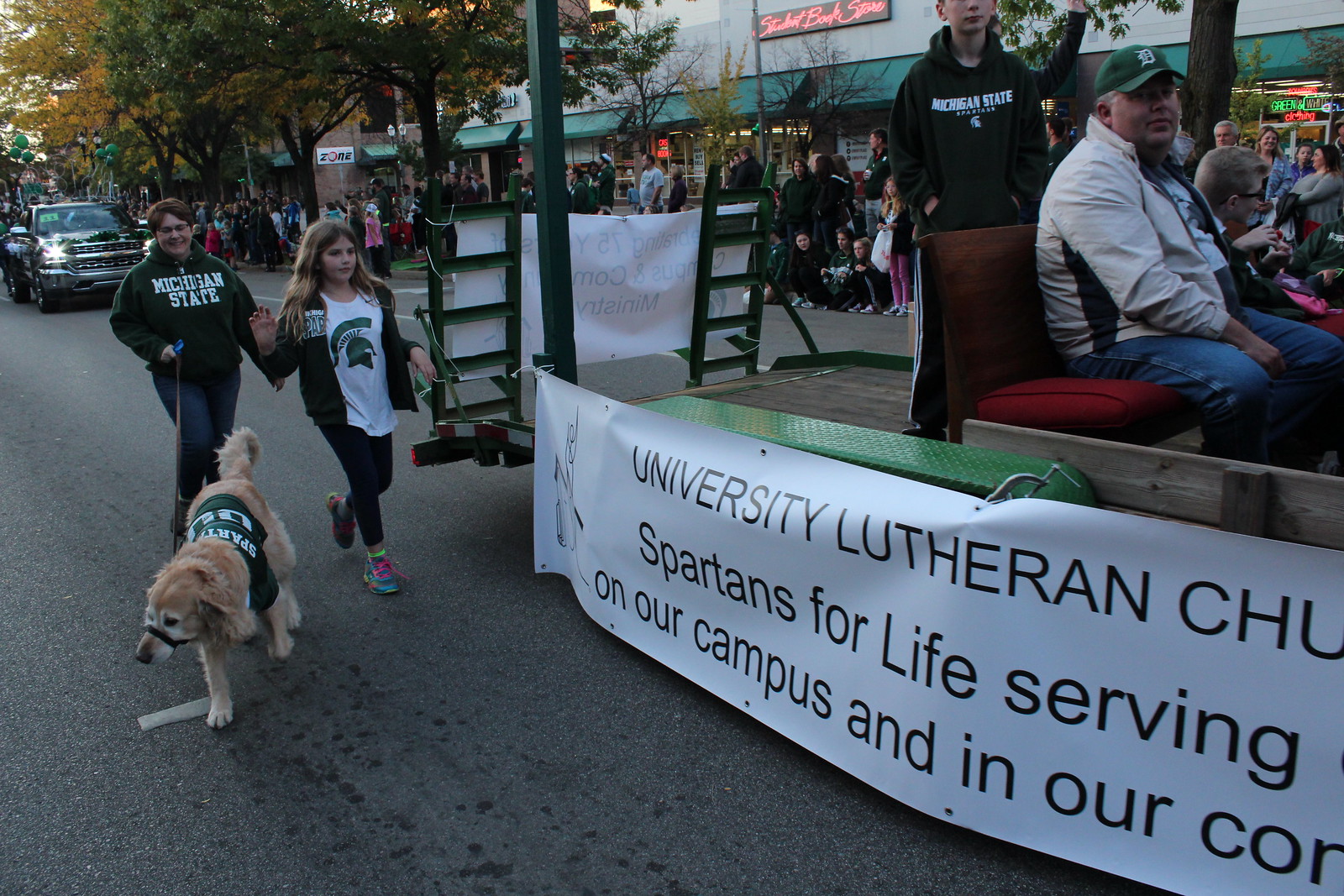This photograph captures a lively parade scene featuring a float from the University Lutheran Church, Spartans for Life. The float is a flatbed truck, adorned with church pews with red cushions, and is bedecked with a large white banner that reads "University Lutheran Church Spartans for Life serving on our campus and in our community" in green lettering. Positioned prominently on a street bustling with activity, the truck is adorned to fit the parade's festive spirit. To the left of the float, a father and daughter duo is walking with their golden retriever, all donning Michigan State gear— the father in a green Michigan State hoodie, the daughter in a white t-shirt with a green jacket, and the dog in a matching green Spartans jersey. Behind the float, a crowded sidewalk lined with storefronts, including one with a sign reading "Student Bookstore," is teeming with spectators, some sitting on the curb. The atmosphere is lively and community-oriented, typical of a college campus event.